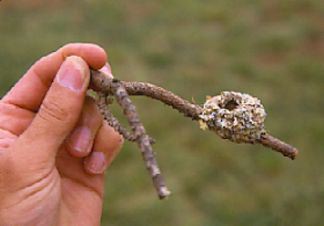In this highly detailed photographic image taken by a nature photographer, the focal point is a white hand, with clean, clipped fingernails, grasping a Y-shaped branch. The branch is held delicately between the thumb and index finger, with the prongs of the Y pointing downwards toward the bottom right-hand corner of the frame. Perched on the tip of the right prong of the branch is a tiny, intricately woven bird's nest, approximately two inches wide, composed of interwoven shades of brown and light brown fibers.

The background features a softly blurred bokeh effect, allowing the viewer to faintly discern the out-of-focus greenery, which likely consists of grass, giving a natural outdoor setting that adds context to the scene without drawing attention away from the main subject. The branch holding the bird’s nest is visually distinct; it is darker in color compared to the left prong, further emphasizing the delicate balance and organic beauty captured within this high-resolution image.